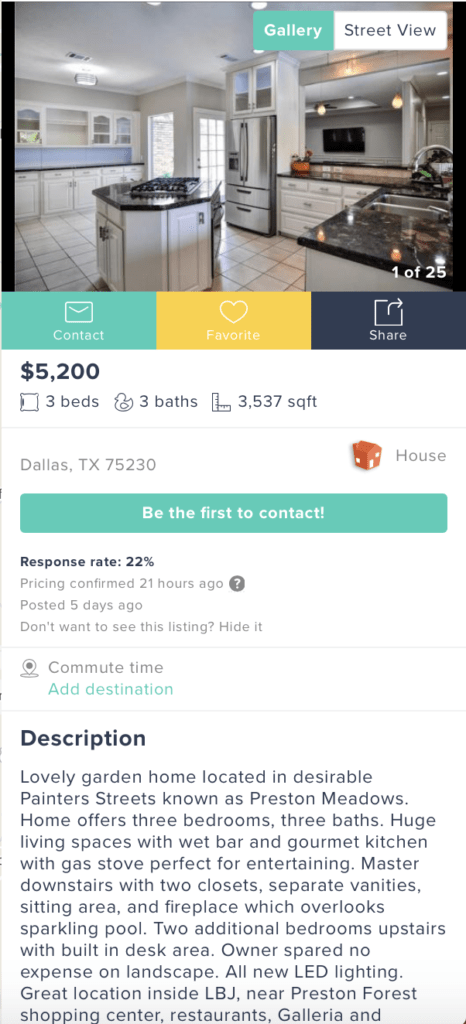The image is a screen capture from a real estate listing on a property website. Prominently displayed at the top is a high-resolution interior photograph of the kitchen. The kitchen features a modern design with an island, white cabinets, white tiled backsplash, and a sleek black granite countertop. A built-in refrigerator and other integrated appliances are visible, complementing the sophisticated look of the kitchen.

Below the image are interactive icons for user engagement: an envelope icon labeled "Contact," a heart icon labeled "Favorite," and a sharing icon. The details of the listing are displayed beneath these icons. The property is listed for $5,200 and comprises three bedrooms and three bathrooms, with a total area of 3,537 square feet. It is located in the 75230 zip code of Dallas, Texas, and is categorized as a house.

An aqua-colored bar invites potential buyers to be the first to contact the seller. Additional text lines provide further details: the response rate is 22%, the pricing was confirmed 21 hours ago, and the listing was posted 5 days ago. There is an option to hide the listing if it doesn't appeal to the viewer.

The screen also provides a feature to select a destination to calculate the commute time from the property’s location. A descriptive paragraph informs about the listing's highlights, describing it as a garden home situated in Preston Meadows. It emphasizes the three bedrooms and three bathrooms, and lists various amenities of the garden home. The listing concludes by mentioning its prime location inside LBJ, near Preston Forest Shopping Center, restaurants, and galleries. Additional information can be accessed by scrolling down.